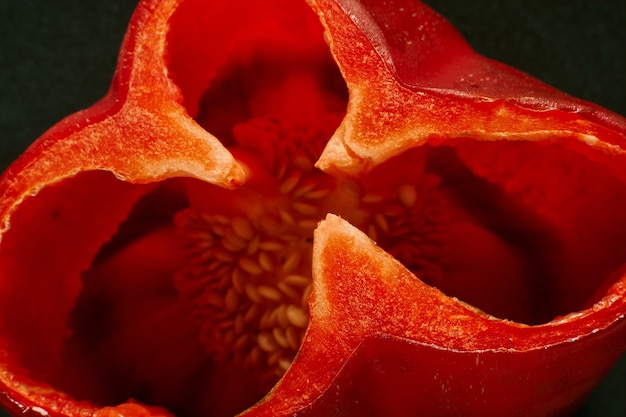This is a sharply detailed close-up photograph capturing the interior cross-section of a red bell pepper, set against a stark black background. The image, framed in a rectangular landscape orientation, reveals the pepper’s trifoil shape at the bottom. The three lobes form circular elements on the left, right, and top, surrounded by a thin red wall that transitions to an orange hue near the cut edges. The deep interior of the pepper is dimly lit, showcasing clusters of yellowish or brown seeds nestled within. Reflections highlight the shiny surface of the pepper’s vibrant red flesh. The hollow spaces inside contrast with the dark void surrounding the pepper, providing a striking visual interplay. There's no text in the image, emphasizing the organic details and the vivid colors of the pepper.